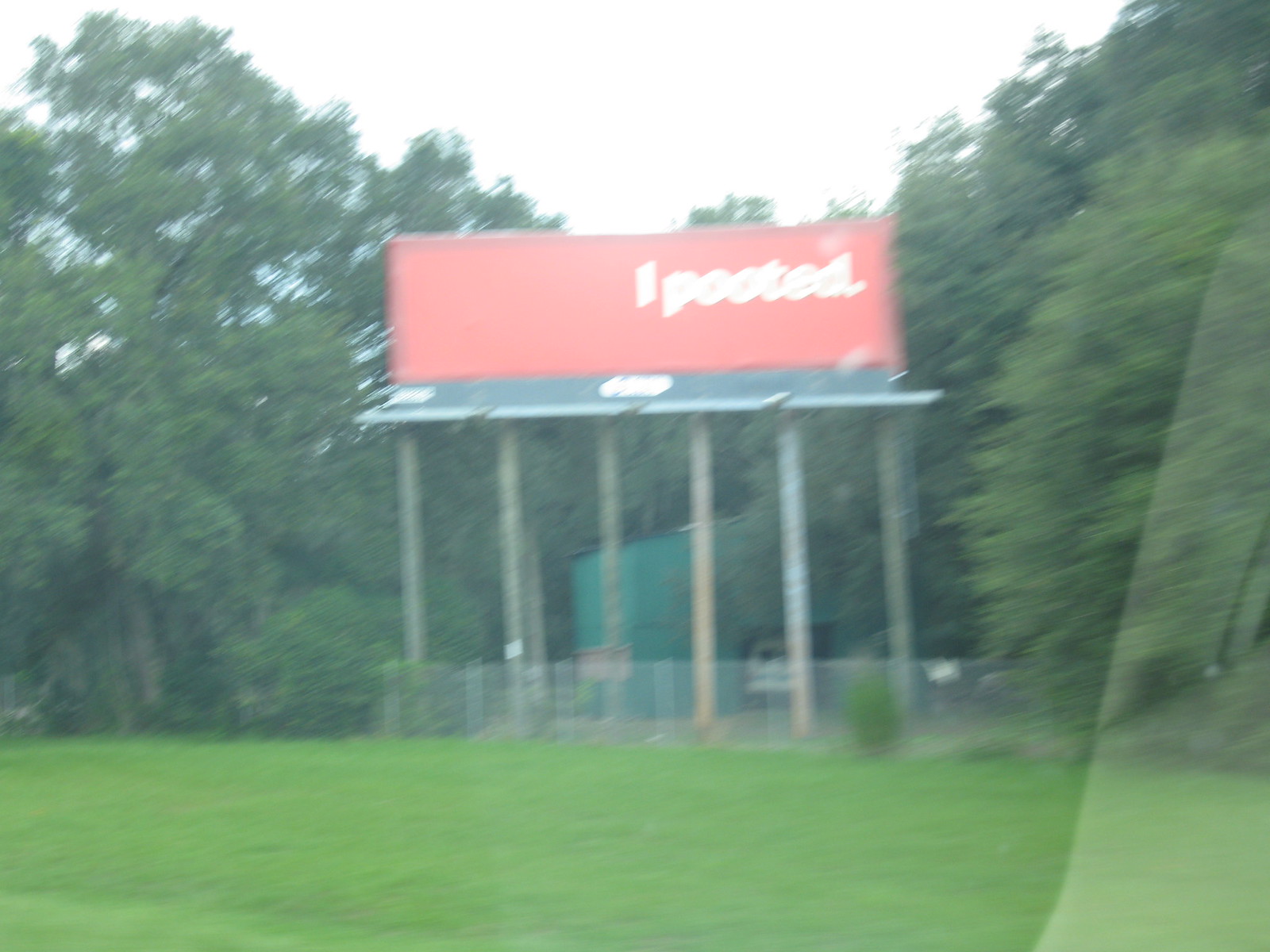This daytime photograph, taken under overcast skies, depicts a billboard seen through the window of a moving vehicle, resulting in a slightly blurry image with visible reflections. The billboard, mounted atop six wooden posts approximately 20 feet above the ground, features the phrase "I pooted" in white font against a red background, located in the upper right portion of the sign. The billboard is set amidst a densely wooded area with numerous trees, with a small green meadow or grassy area in the foreground between the photographer and the billboard. The sky, obscured by the overcast conditions, appears to be an indeterminate whitish color.